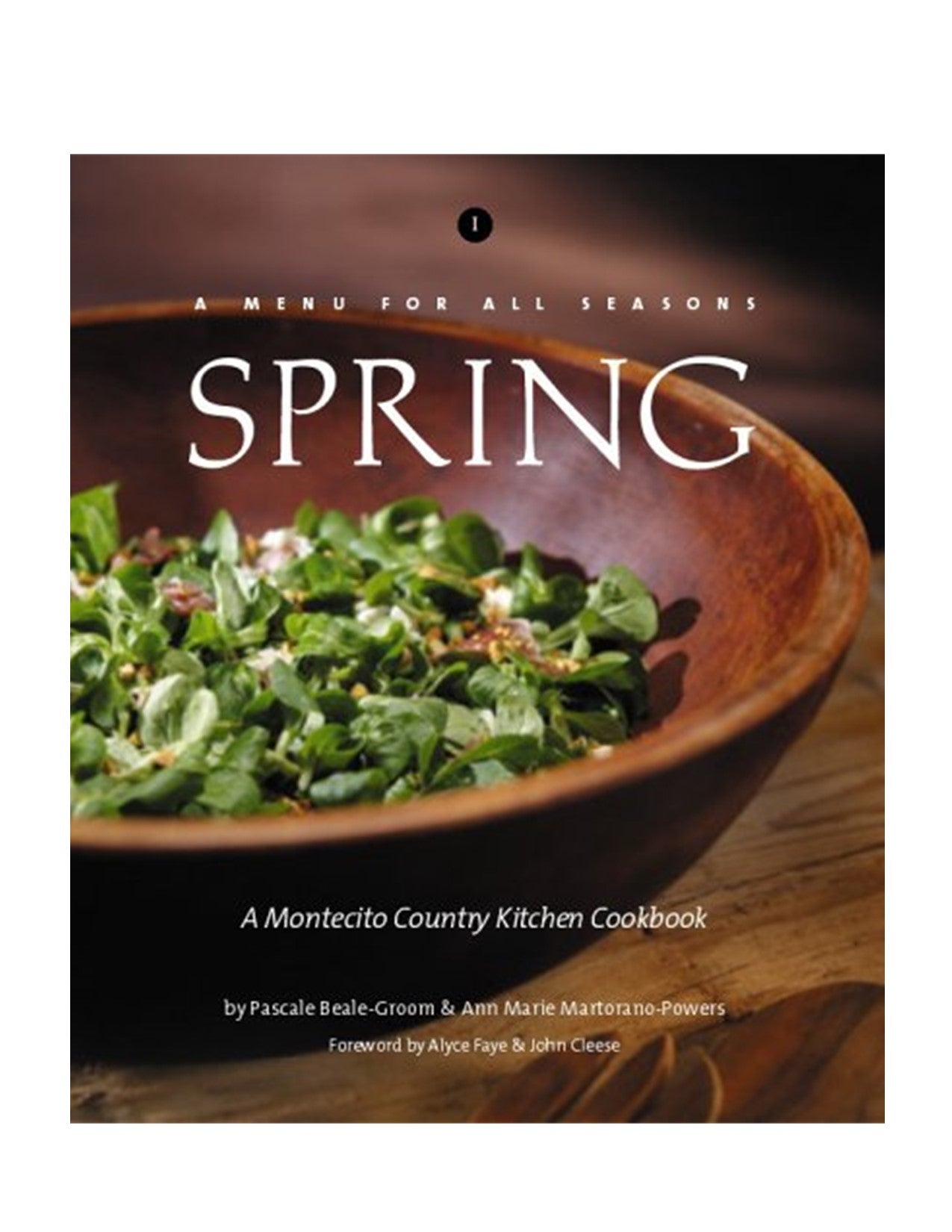This color image is the cover of a cookbook titled "A Menu for All Seasons: Spring." The title is displayed prominently in white text at the top and center of the image. Beneath the title, in smaller white text, it reads "A Montecito Country Kitchen Cookbook by Pascal Beale-Groom and Anne-Marie Martorano-Powers," followed by "Foreword by Alice Fay and John Cleese."

The focus of the photograph is a wooden bowl filled with fresh salad greens and small brown bits, possibly seeds or croutons. The bowl, which is a darker reddish-brown, sits prominently on a light brown wooden table or countertop, distinguished by its dark brown grain. At the bottom of the image, a wooden fork and serving spoon are partially visible, adding a rustic touch to the aesthetic.